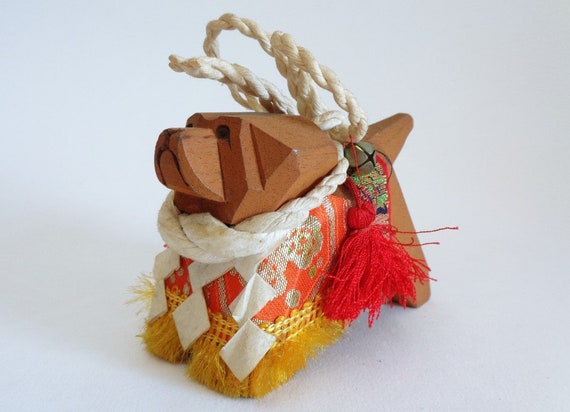This image captures a detailed depiction of a crafted wooden dog, possibly intended as a Christmas ornament. The dog, carved from wood and set against a solid white background, stands at an angle with its face towards the bottom left. The dog has expressive black eyes and several distinguishable features, including ears, a nose, a mouth, and a tail. Around its neck, there is a woven rope that loops in a pretzel-like fashion, and it continues up behind its head. The dog is adorned with a colorful cape-like garment that features a coral material with a silver flower on the front body. This garment also has a gold trim along the bottom edge and yellow fringe on the arms. Additionally, there are red tassels hanging off the back, accompanied by a small silver bell. The overall design and intricate decorations suggest a vaguely oriental theme, adding a unique charm to the piece.